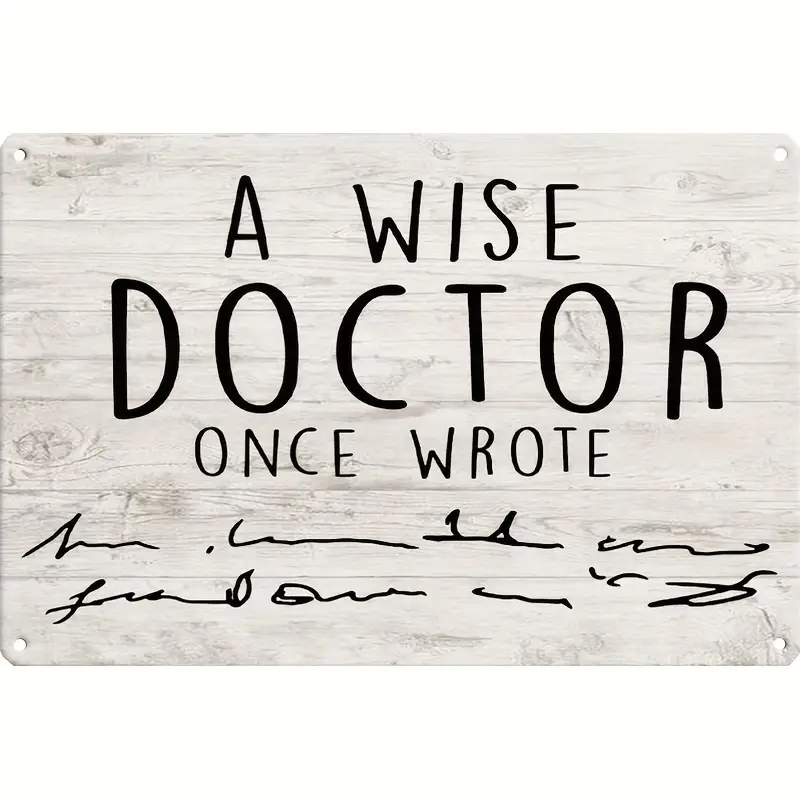The image showcases a rectangular board with a faux wood grain texture, appearing gray in color, against a white background. The board features clearly legible text that reads, "A wise doctor once wrote," followed by two lines of scribbled, unintelligible handwriting, humorously mimicking the notoriously poor handwriting of doctors. Each of the board’s four corners contains what appears to be a nail or screw, giving the impression that it is affixed to the background. The board's edges are curved, contributing to its decorative appeal. This piece of art humorously plays on the stereotype of doctors' illegible writing and is designed to be either a wall hanging or a decorative sign.